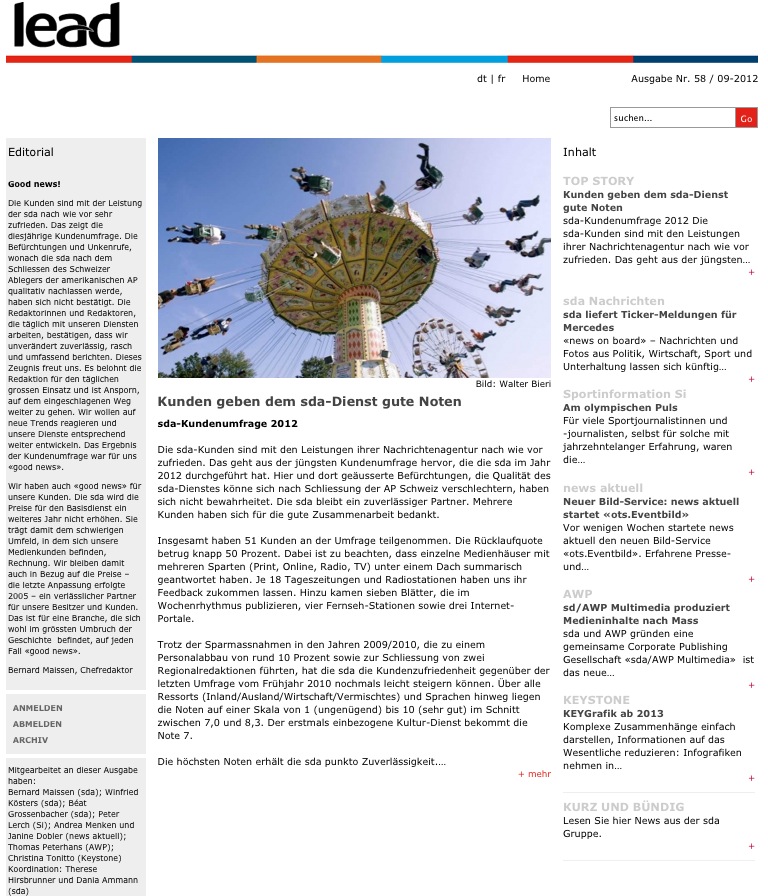The image depicts a German webpage or periodical titled "LEAD" prominently displayed in the top left corner. The date "9-20-12" is seen on the top right, along with the words "EDITORIAL" and "GOOD NEWS!" centrally placed. The page showcases a visual of an amusement park ride in the middle, featuring people seated on chairs suspended by strings from a spinning structure, with a distant Ferris wheel visible in the background. Below the image, the caption reads "BALD WATER BE AIRY." The article appears to discuss topics including customer satisfaction, editorial insights by Bernard Meissen, and high marks received by the SDA service in 2012, derived from a detailed survey with a 50% response rate. It emphasizes the reliability of the SDA service across multiple media platforms like print, online, radio, and TV, despite prior austerity measures and staff reduction. This detailed and translated overview provides context for understanding the essence of the webpage.